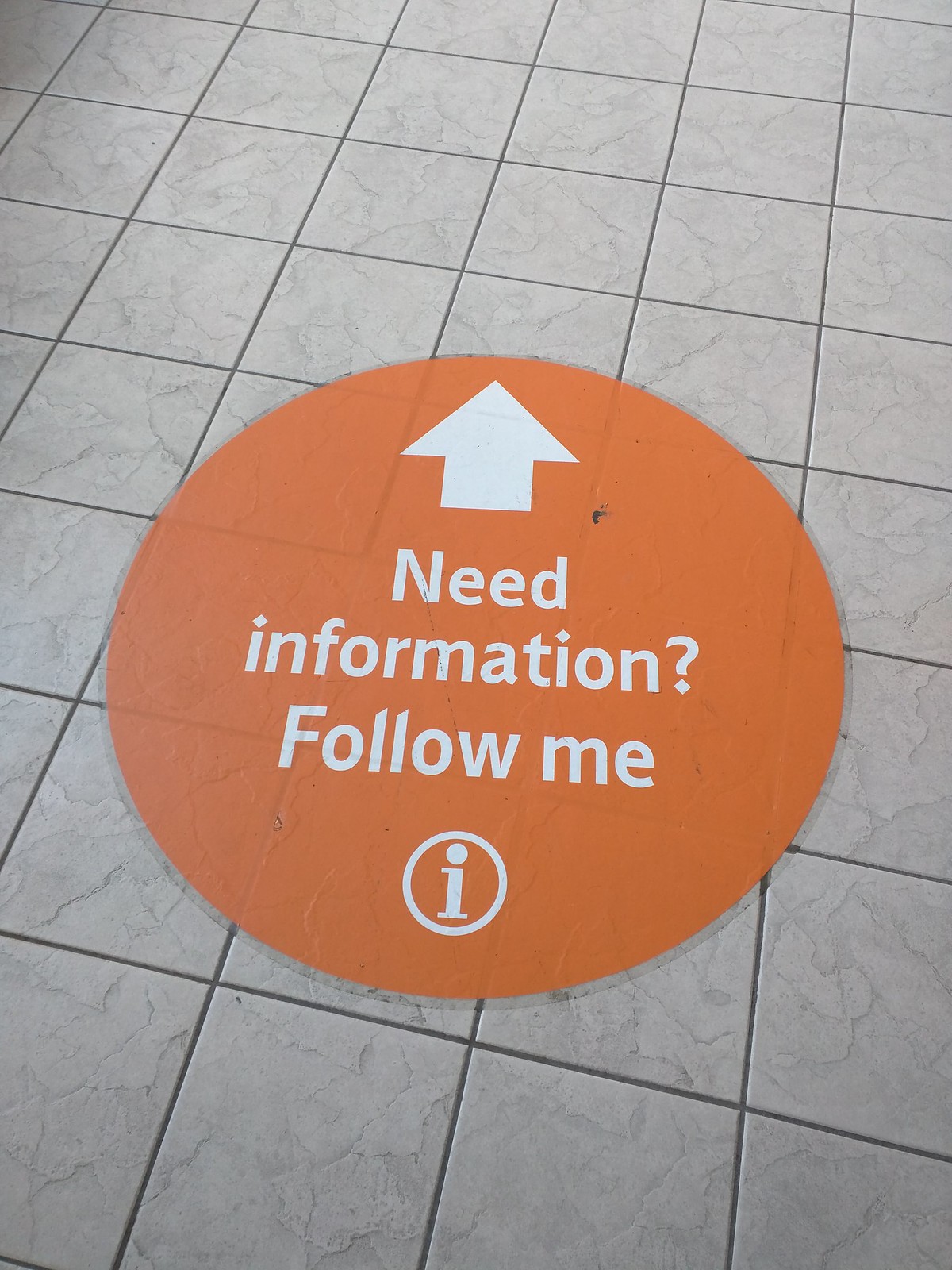The image displays a vertically aligned, rectangular picture predominantly featuring a light gray, marbled tile floor with small, neatly aligned square tiles and darker gray grout lines. The visually striking centerpiece of the image is a large, circular, orange mat or sticker, which occupies a space equivalent to a three-by-three grid of the tiles. This circular element has a white up arrow and accompanying white text that reads, "Need information? Follow me," with a lowercase "i" encircled in white beneath it. The surface of this sign exhibits some scuffs and scratches, indicating it has been frequently walked on. The overall scene is characterized by the juxtaposition of the clean, geometric tile arrangement and the vibrant, slightly worn informational marker.